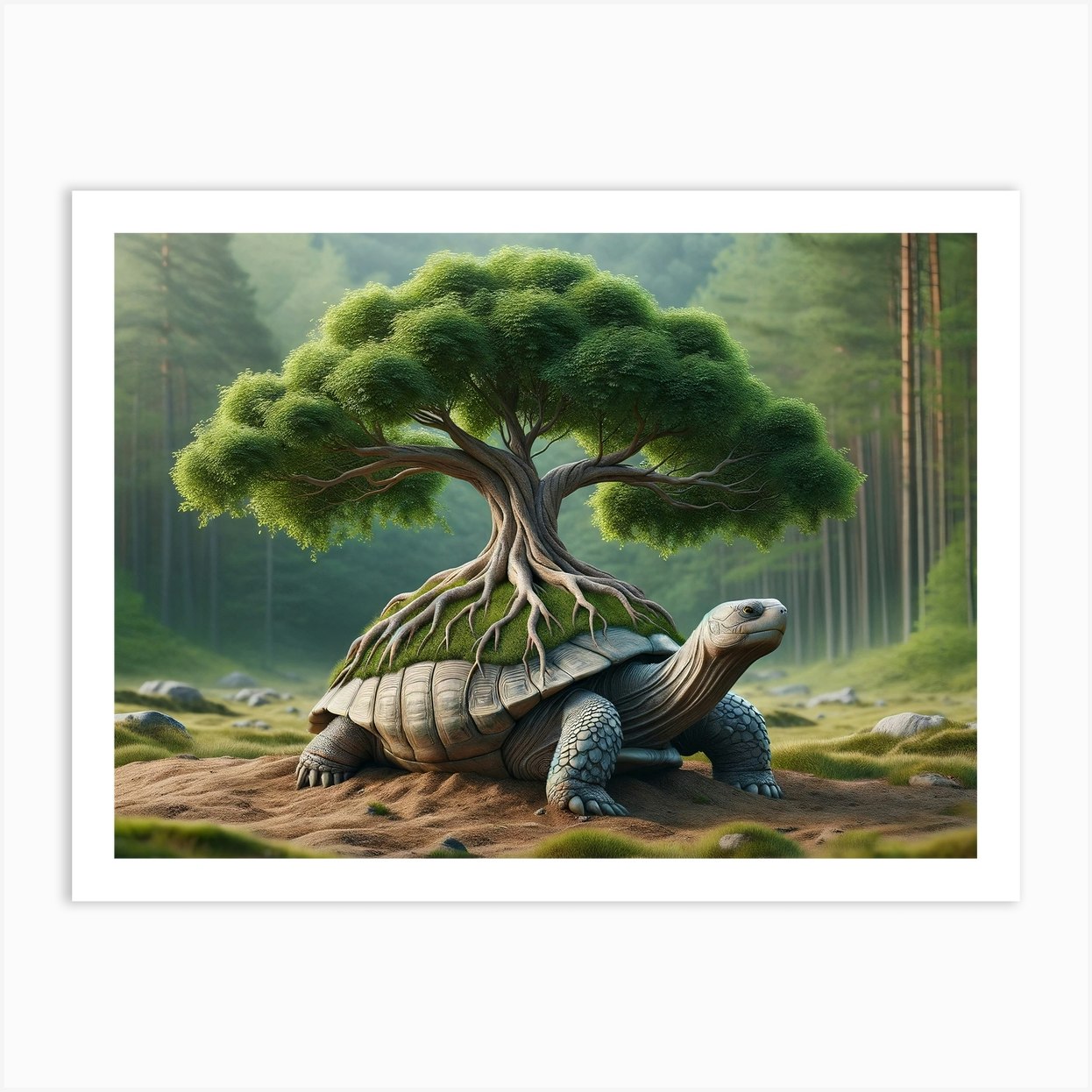This is a digital print or lithograph of a whimsical painting, presented as a wall hanging with a white border around it, displayed on a white wall. The central focus of the artwork is a determined-looking tortoise, depicted in a three-quarter view, crawling on light brown dirt. The tortoise, predominantly grayish-brown in color, is shown with its head up and legs extended. On top of its shell, which is slightly slanted towards the back, grows a fully-formed miniature bonsai tree with thick branches, brown trunk, and a mix of hunter green and light green leaves. The shell is also adorned with lush green grass, through which the tree's roots are visible. In the background, there is a blurred depiction of a forest with tall, muted trees and bushes, rendered in various shades of green and brown, enhancing the focus on the tortoise and its curious botanical burden. The image has a serene, yet surreal quality, and appears to be available for purchase online.